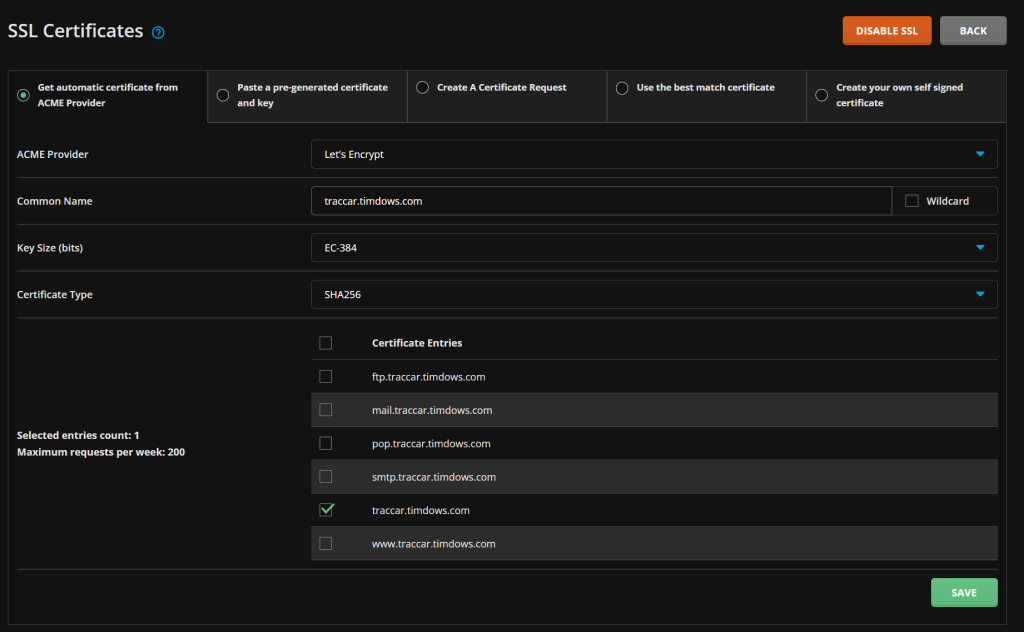Image Description: 

The image features a user interface with a black background. In the upper left corner, "SSL Certificates" is written in a blue outlined font, accompanied by a blue-outlined question mark inside a circle. The upper right corner of the image contains two buttons: an orange button with white text reading "Disable SSL," and to its immediate right, a gray button with white text reading "Back."

Beneath "SSL Certificates," a green-highlighted option is marked as clicked, reading "Get Automatic Certification from Acme Provider." There are several other tabs aligned in a horizontal strip across the top, each representing different options: "Paste Pre-Generated Certificate and Key," "Create a Certificate Request," "Use the Best Match Certificate," and "Create Your Own Self-Signed Certificate." None of these tabs are currently selected.

On the left side of the main content area, a section with labels and input fields is visible. The labels include "Acme Provider," "Common Name," "Site," "Key Size," "Bits," and "Certificate Type." To the right of each label are corresponding input fields, most of which are dropdown menus:

- The dropdown menu under "Acme Provider" is set to "Let's Encrypt."
- The "Common Name" field, which is not a dropdown, displays "traccar.timdows.com." Adjacent to this field is an unchecked box labeled "Wildcard."
- Under "Key Size," the field displays "EC-384" with a dropdown menu option.
- The "Certificate Type" field is set to "SHA-256," also with a dropdown menu option.

The layout suggests a form-like interface designed for managing SSL certificates, with specific focus on options provided by an Acme provider.